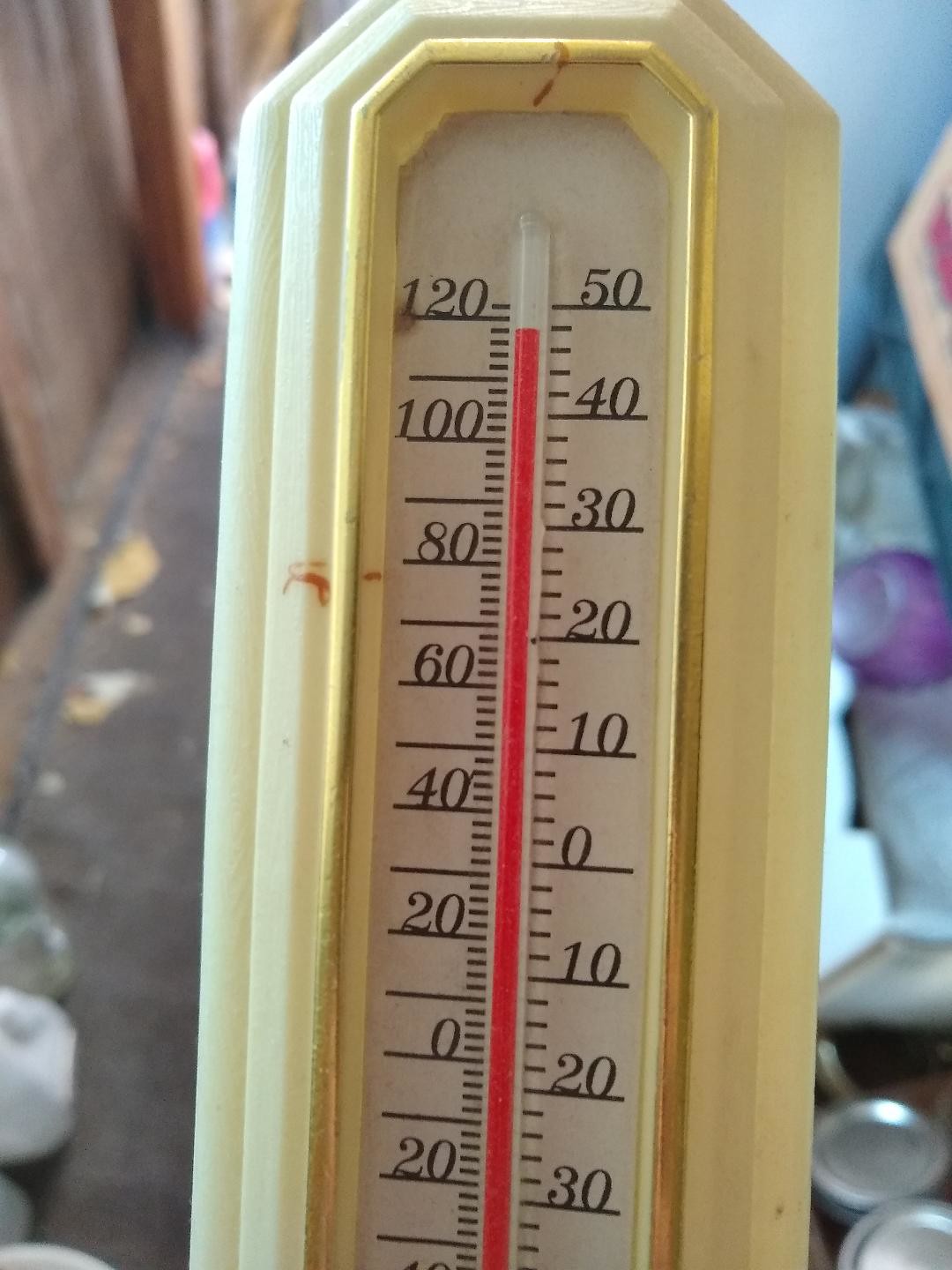This is a detailed photograph taken in portrait mode of an outdoor thermometer, captured in what appears to be an alleyway or possibly a garage setting. The floor in the background is composed of rough concrete, and to the lower left corner, several white plastic bags are resting haphazardly. In the upper left section of the image, a plywood section of wall is visible, anchored by a sturdy wooden post. The right side of the frame features a blue wall, alongside the edge of what looks like a folded white TV tray table. Below this table, numerous silver cans are neatly stacked. Dominating the center right of the image, within a white box turned on its side, is a striking purple, glass-like round object. The thermometer itself is framed in an ivory-colored casing with a slightly yellowish tint and angled sides. The central area of the thermometer is white, displaying black numeric markings. The red mercury inside indicates a sweltering temperature of 119 degrees.